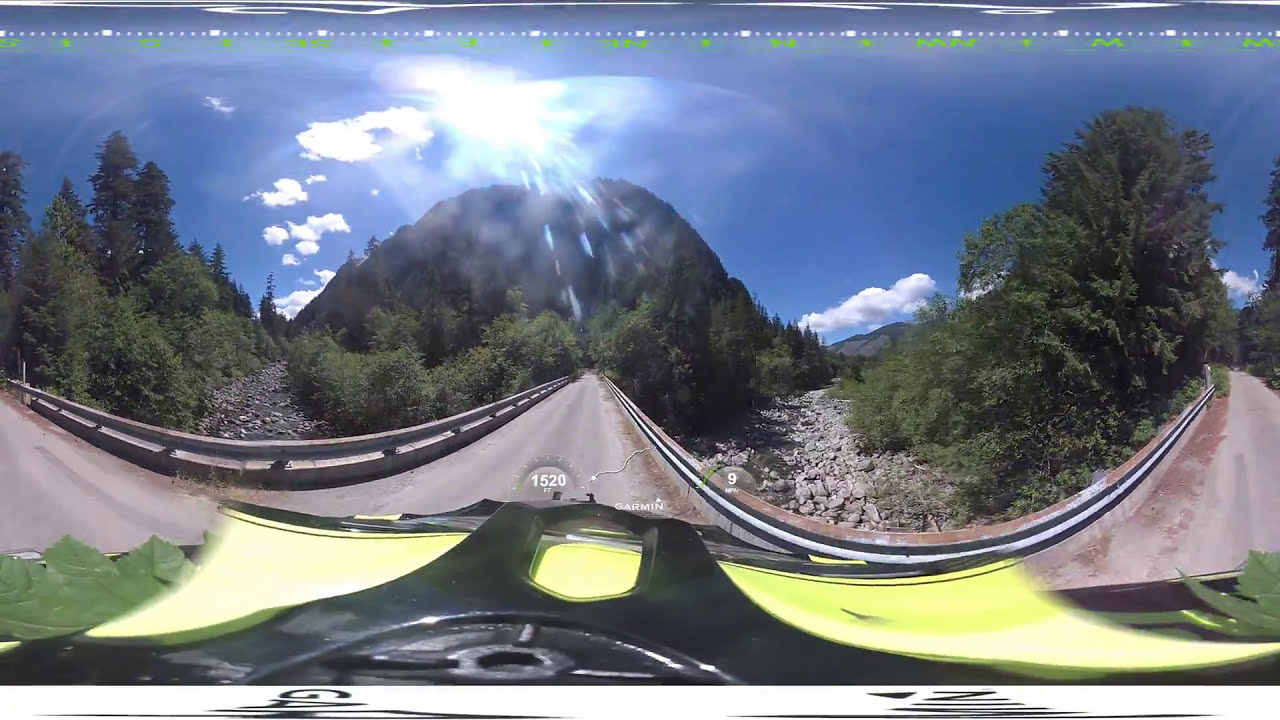A wide-angle photograph captures a deserted road, viewed from the perspective of someone driving a vehicle, possibly a motorcycle or a car. The curved and distorted appearance of the image suggests it might be a 360-degree shot. The road, flanked by metallic guardrails, runs towards a towering, tree-covered mountain under a vibrant blue sky with a few fair-weather clouds. A bright sun peeks through the clouds, casting light across the scene. To the right, a deserted road branches off, seemingly leading straight down, while to the left, a rocky outcrop descends into a nearly dried-up riverbed strewn with rocks, surrounded by tall pine trees and smaller bushes. Text overlay on the image reads "1520 feet, Garmin, 9 MPH." Additionally, there are green markings and some white dots, indicative of the camera's settings or a heads-up display, confirming the photographic origin of the scene.